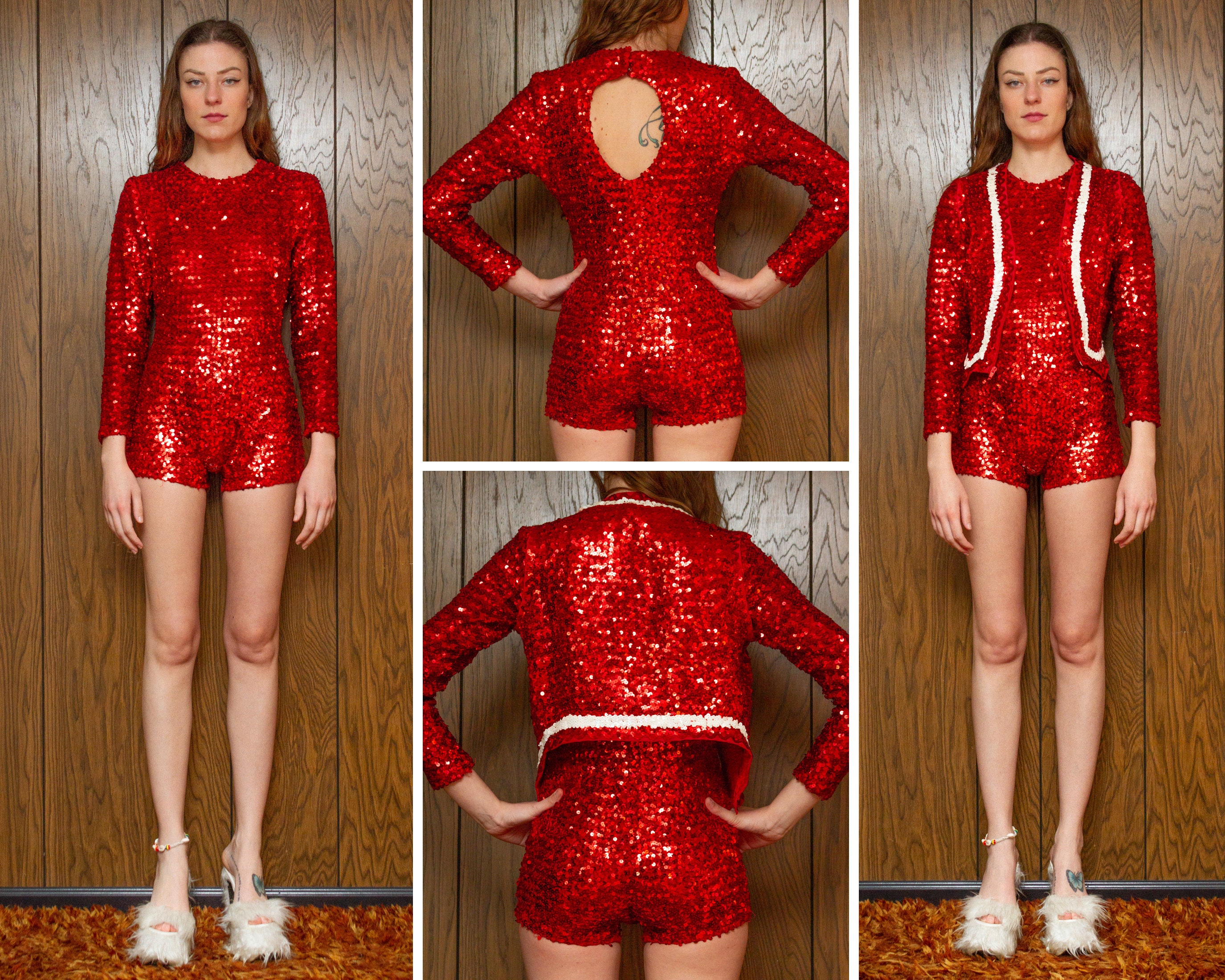The image features a sequence of four photos of the same woman, showcasing her in a sparkling red one-piece outfit that extends to the top of her thighs, revealing her bare legs. She is wearing high heels adorned with white fur, and in all the photos, she stands on a brown shaggy carpet that meets a black strip against a background of wooden panels with visible grain and darker brown lines.

The first and last images on the left and right, respectively, depict her standing in the red outfit in front of the wooden panels. In the leftmost image, she wears an ankle bracelet on her right ankle and poses with the full outfit. In the rightmost image, she has modified the outfit by adding a vest with white stripes on the lapels.

The central images provide a detailed view from behind. The upper image shows her back, revealing a tattoo and the original outfit without modifications. The lower central image features her from the same angle but now wearing the vest with white strips around the collar and bottom, matching her shoes.

Overall, the series appears to document a "before and after" transformation of her outfit, maintaining consistent elements like her ankle bracelet, fluffy white high heels, and the wooden panel backdrop.